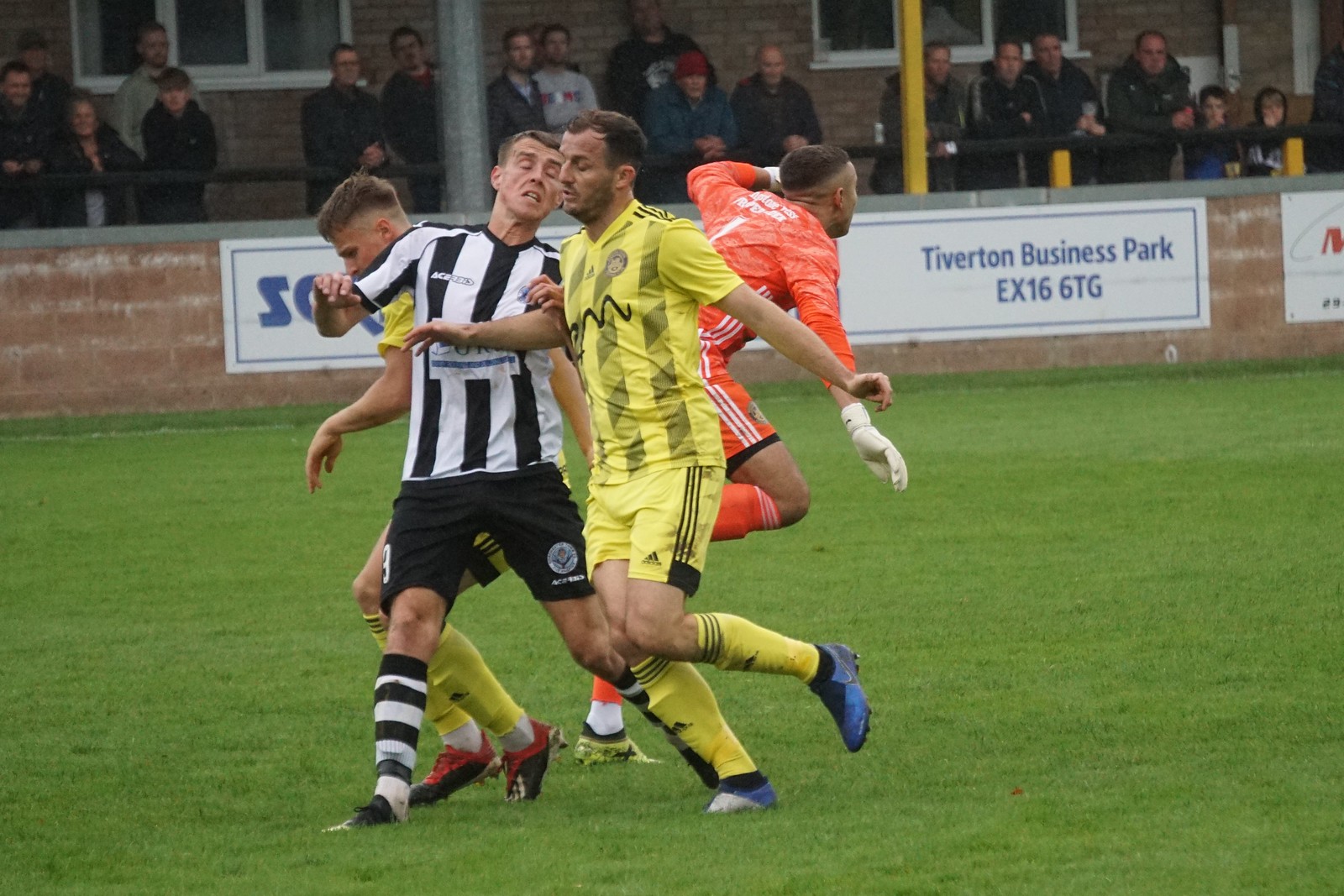In this detailed image of a European football game, a dynamic scene unfolds on a lush, green pitch. At the center of the action are four key figures: two players clad in yellow and black jerseys, another in an orange and white uniform, and a referee sporting a black and white striped jersey with matching socks. The players appear to be clashing mid-field, coinciding with the referee who seems caught in the midst of this chaotic moment, possibly trying to intervene or being inadvertently knocked by the momentum of the players. Surrounding the field is a brownish wall adorned with various advertisements, one notably saying "Tiverton Business Park EX16GTG". Behind this wall, spectators are gathered, bundled up in long-sleeved coats and hats against the cold, watching from a balcony against a brick backdrop. The sky is overcast, adding to the overall chilly atmosphere.